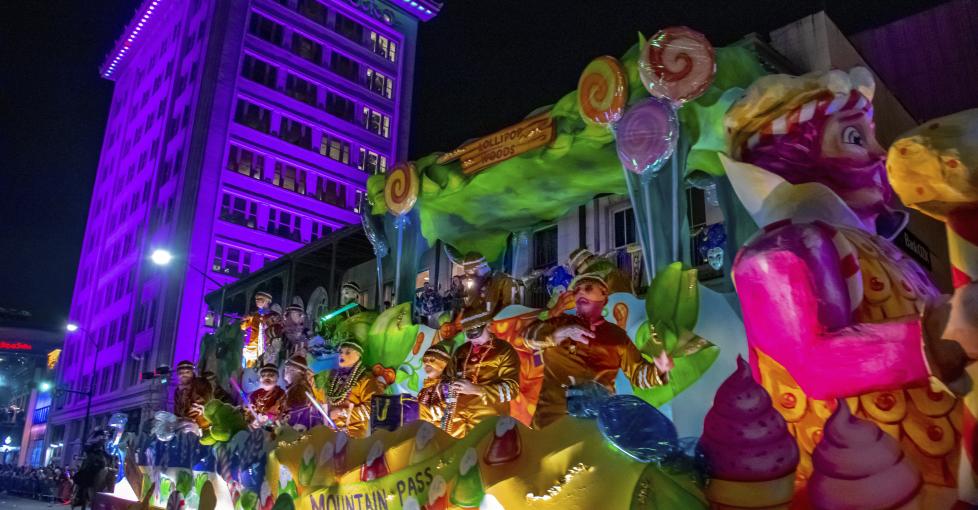This image depicts a vibrant, night-time parade likely set in a New Orleans-esque setting. Dominating the scene is a large, colorful float, adorned with candy-themed decorations reminiscent of a Willy Wonka-esque or 70s psychedelic art style. The float is festooned with oversized lollipops in various colors, including large purple, orange-yellow, and red-pink swirled designs. A prominent green banner on the side reads "Mountain Pass," and another sign at the top of the float declares "Lollipop Woods," adding to the whimsical, fantastical theme.

At the front, a massive paper-mâché figure, a man with pink hair and a pink beard, dressed in pink and adorned with candy canes and cupcakes, holds a large candy cane. Beneath the float, men in yellow outfits toss candy to the crowd. The float and its details are dramatically lit from below, casting vivid colors against the dark, starless sky.

In the background, the towering purple-lit skyscraper and a smaller, older-looking building reflect the architectural styles seen in New Orleans. Throngs of spectators line the street, some stacked or standing on the side of the road, further suggesting a lively parade atmosphere. This well-lit and colorful scene captures the jubilant, imaginative spirit of a festive night parade.